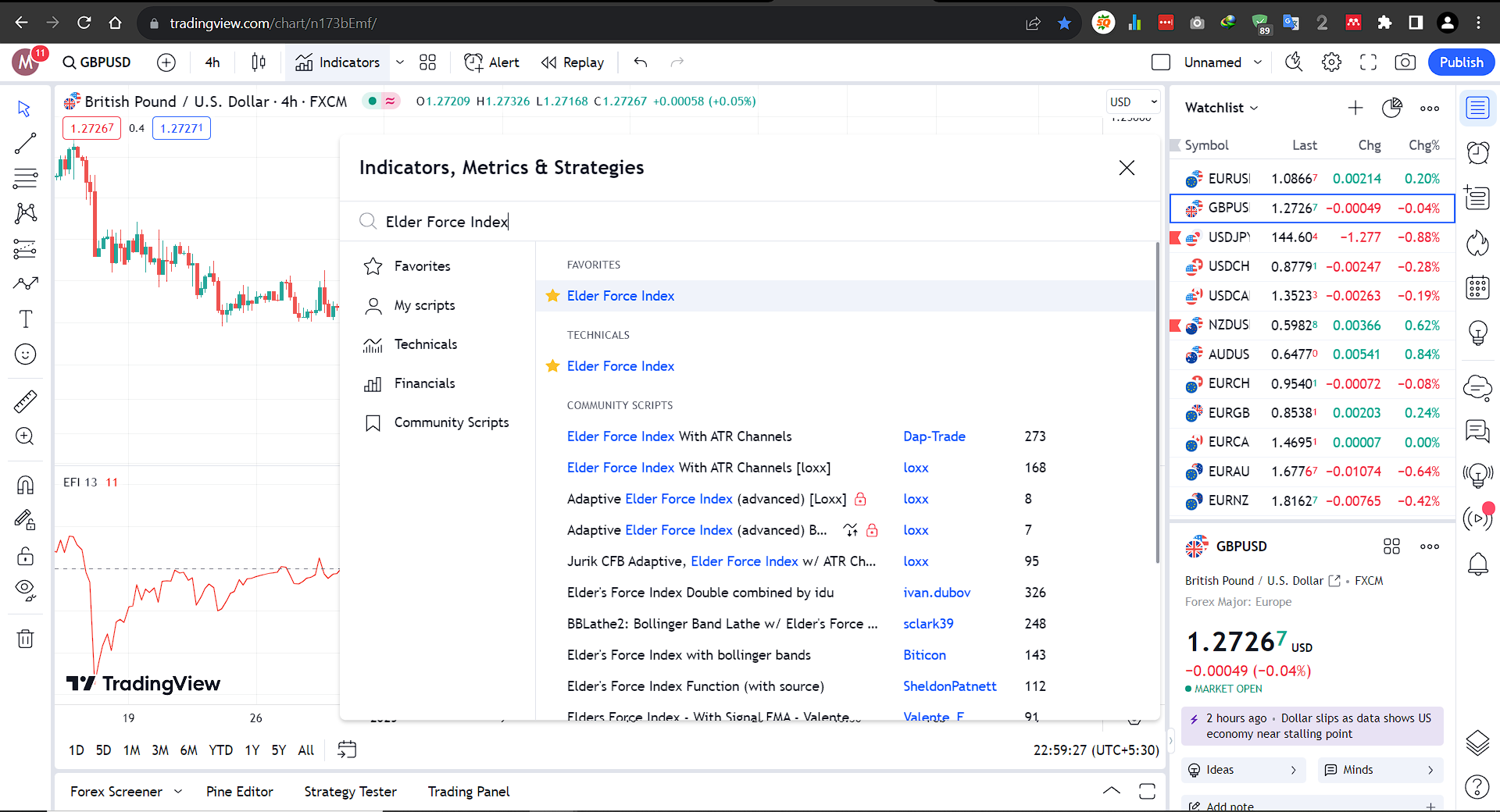The image is a screenshot from the TradingView platform, displaying the British Pound to US Dollar (GBP/USD) exchange rate. The main section of the image features a detailed graph with blue and red lines indicating price movements over time. Below this graph, there's another graph represented by a solitary red line. 

To the right of the graphs, there's a sidebar titled "Indicators, Metrics, and Strategy," which includes options such as "Elder Force Index," "Favorite," "My Script," along with others categorized under technical, financial, and community scripts. This sidebar also contains some blue and black text with terms related to the Elder Force Index and other indicators.

At the very top of the image, there's a black taskbar containing over a dozen miscellaneous icons. Below the graphs, there's a list displaying various stock numbers and their corresponding prices.